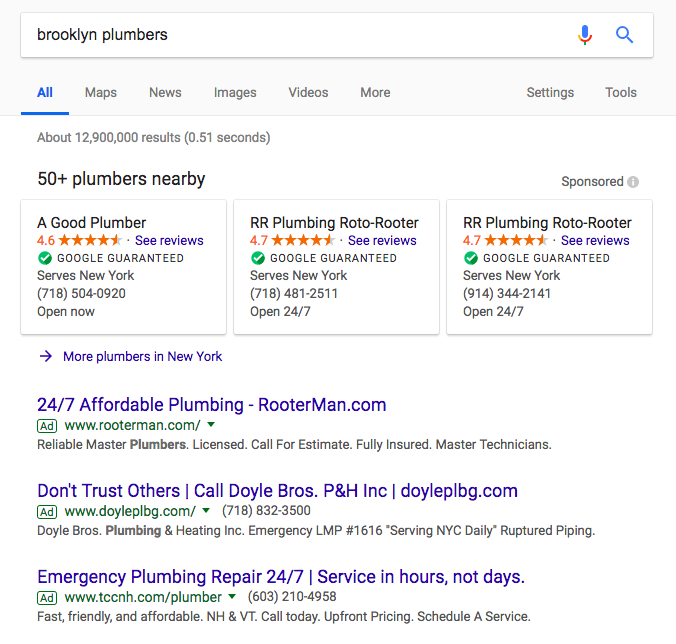The image appears to be a screenshot of Google search results for "Brooklyn plumbers." At the top, there is a microphone icon next to the search bar, indicating that voice search may have been used. The background is predominantly white, in line with Google's typical search results layout. 

The search results showcase a list of plumbing companies in Brooklyn, each accompanied by user ratings. The top entries include companies such as "A Good Plumber" and "Roto-Rooter Plumbing & Water Cleanup," both highly rated with averages of 4.6 and 4.7 stars, respectively. The ratings are displayed in orange for visibility.

A notable feature in the search results is the "Google Guaranteed" badge, indicating that these businesses have met certain criteria set by Google, providing an extra layer of trust. The text is predominantly black, with company names in blue, and occasional ads highlighted with green text. Overall, the design is simple and clean, consistent with Google's conventional search results page.